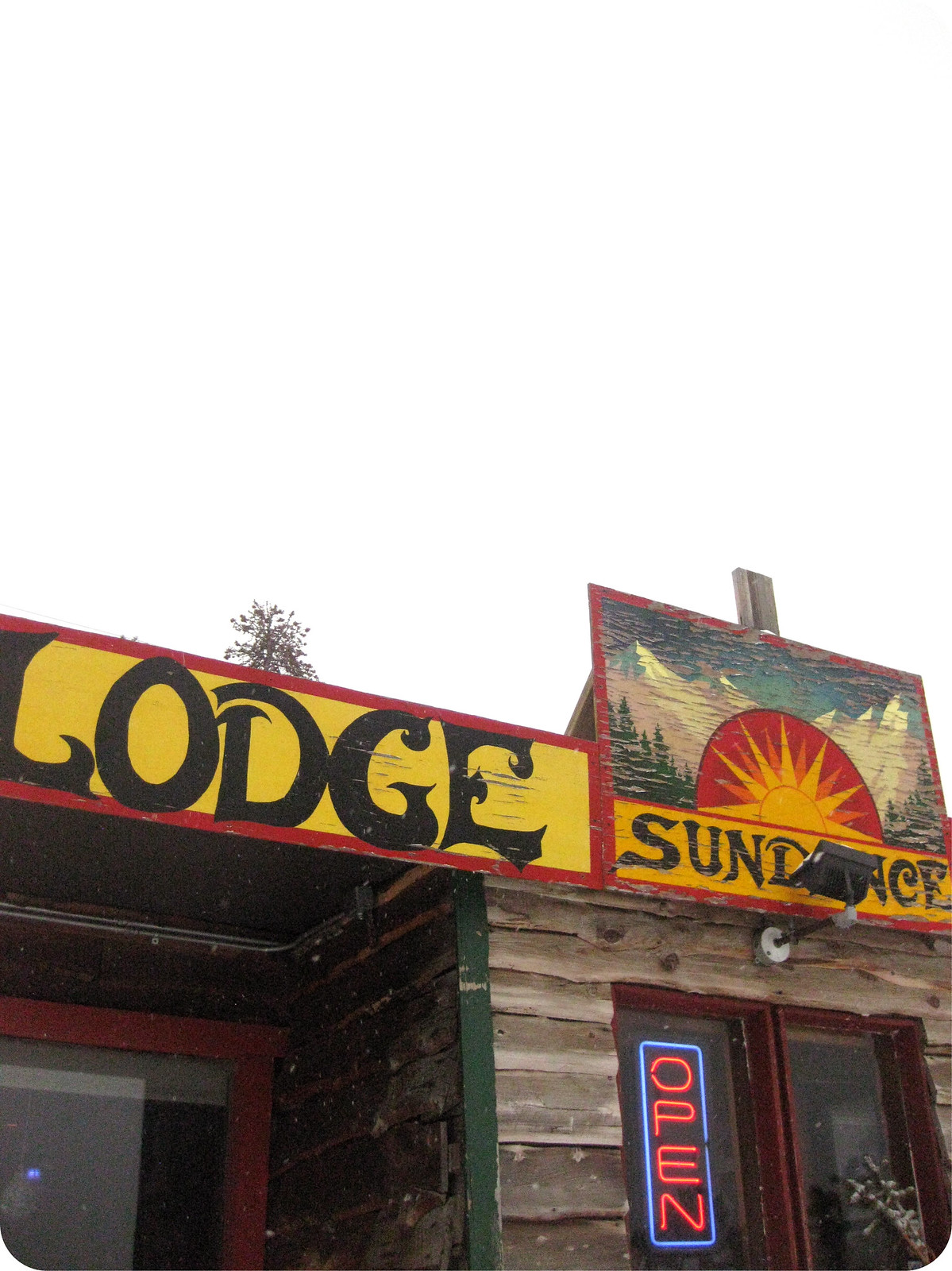This is a detailed photograph capturing the front of a rustic lodge named "Lodge Sundance." The structure is constructed primarily of aged wooden planks, evident by the peeling paint that adds to its weathered charm. The photo, taken from a low angle, accentuates the lodge against a nearly indistinguishable, light sky, revealing just the faint outline of a distant tree.

Prominently displayed at the top of the building are two weathered wooden signs. The first sign reads "Lodge" in thick, black lettering with a red trim on a yellow background. The adjacent sign states "Sundance" in black type atop an aged yellow backdrop, featuring a stylized sun logo and a hint of mountains and trees, suggesting a scenic locale like Colorado, Idaho, or Utah.

Below these signs, there's a red and blue neon "Open" sign mounted on the wood. This sign is centrally located near a door at the bottom of the image, indicating that the lodge is welcoming visitors. The overall color palette of the scene includes natural browns, greens, yellows, reds, blacks, and whites, enhancing the lodge’s inviting yet time-worn appearance.